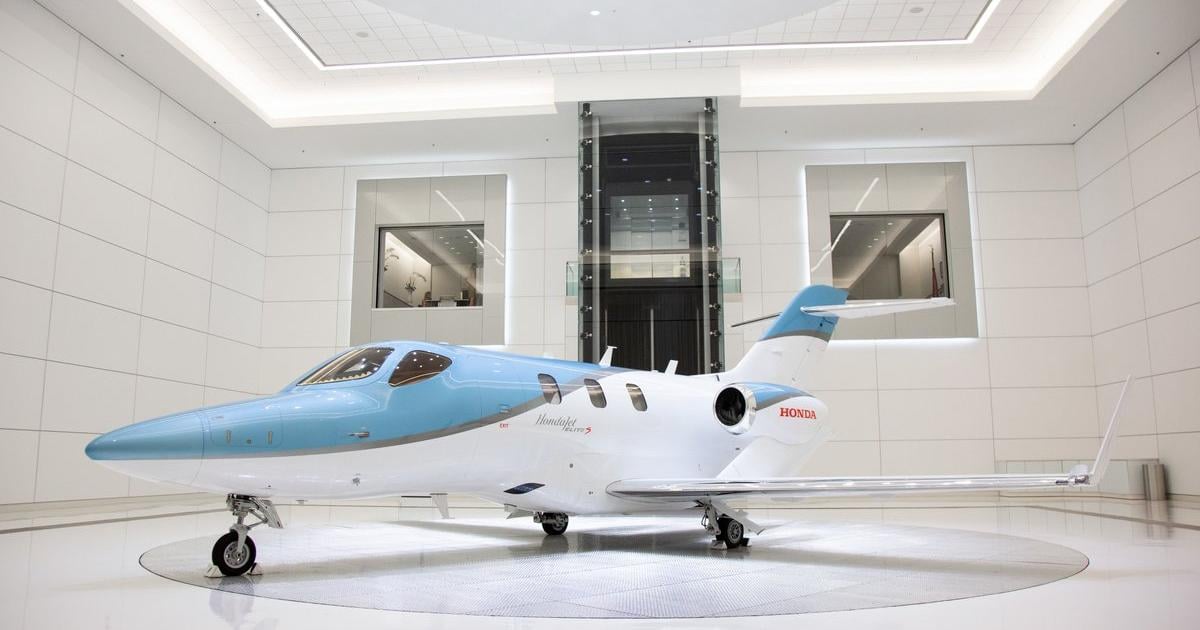This photograph captures a sleek, small jet airplane prominently displayed in a pristine, white room that resembles a museum gallery. The room features a white ceiling, shiny white floor, and large white panels on the walls. At the back, there's a black entrance door topped with a window, flanked by two larger windows that let in ample natural light. Above, a glass ceiling further illuminates the space. The main attraction, the airplane, is mostly white with distinct light blue paint wrapping from the nose, over the cockpit, and extending halfway along the top, blending into the wing area. It is equipped with two engines mounted at the rear, a pointy nose, and three landing gear wheels. The jet has three small passenger windows on the side, and a prominent red Honda logo near the tail. The aircraft is positioned on a gray circular platform, emphasizing its polished and modern appearance.